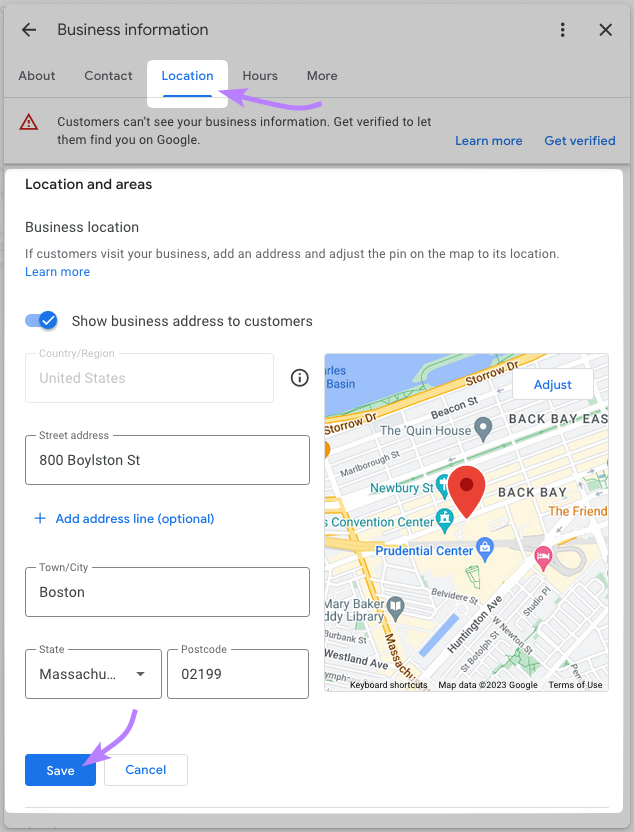The image appears to be a screenshot of a Google business location settings page, detailed as follows:

At the top and bottom of the page, there are purple sections. In the top left, there's a left arrow adjacent to the text "Business Information." Next to it, a grey section displays options such as "About" and "Contact."

In the center area, there is a white square with blue text labeled "Location." 

To the right of this, additional information about the business location is provided, featuring a message within a purple arrow and a red triangle icon stating: "Customers can't see your business information. Get verified to let them find you on Google. Learn more. Get verified."

Below the main heading, it says "Location and Areas" followed by "Business Location," with an instructional message: "Your customers visit your business. Add an address to place a pin on the map for its location. Learn more."

There's a toggle setting labeled “Show Business Address,” with various input fields for address details including:
- Name of the state: Massachusetts
- City: Boston
- Address: 800 Boisland Street
- Postcode: 02199

A blue square with an arrow icon appears next to "Save" and "Cancel" buttons. At the top, there's an "Out of Order" notification next to "Star Road, Bing Street, the Quinn House." A red pin marks a location on a map centered in the image.

In the bottom left, the "Mary Baker Library" is shown, while in the bottom right, there is text reading "Hometown." Beneath the map, options for "Keyboard Shortcuts," "Map Data" from either Google, and "Terms of Use" are visible.

The overall context suggests this is part of a Google My Business settings interface aimed at managing a business's location details and verifying its information for public visibility.